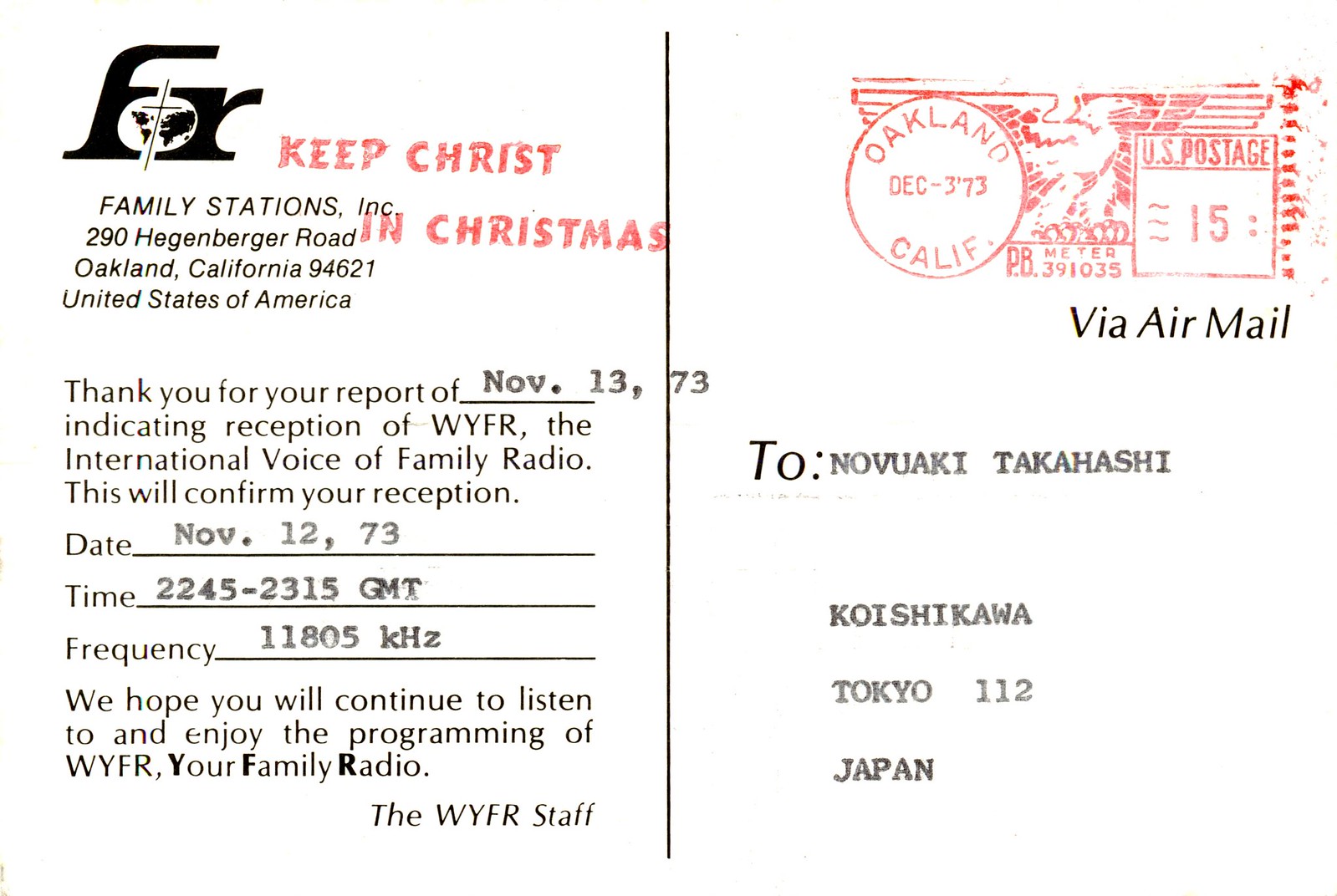The photograph displays the back of a postcard from Family Stations, Inc., located at 290 Hegenberger Road, Oakland, California, 94621, USA. Prominently featured is a red stamp urging to "Keep Christ in Christmas." The postcard is addressed via airmail to Nobuaki Takahashi in Japan. The top left of the card confirms receiving a report dated November 13, 1973, indicating the reception of WIFER, the International Voice of Family Radio. The reception details include the date, November 12, 1973, time from 22:45 to 23:15 GMT, and frequency 11805 KHC. The message expresses appreciation for listening and hopes the recipient will continue to enjoy WIFER's programming. The correspondence highlights a heartfelt connection through international radio communication.